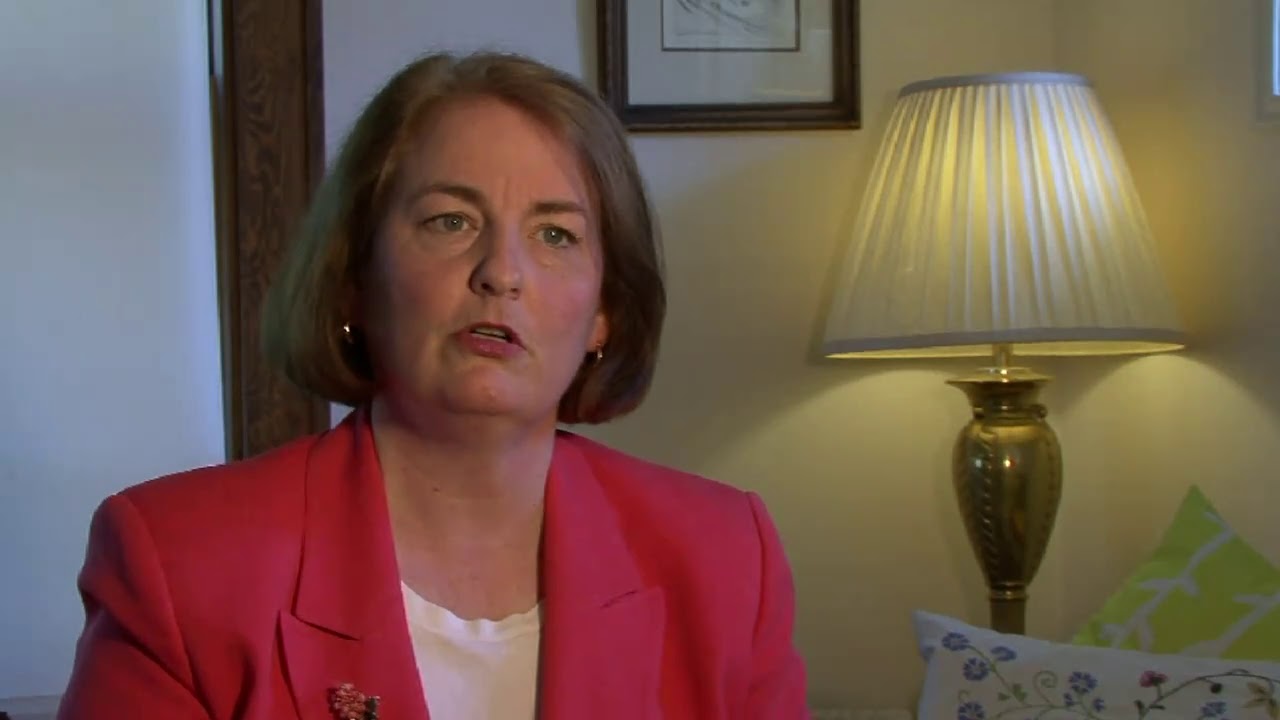In this image taken indoors, likely during an interview, a woman in her mid-40s to 50s is the focal point. She sits slightly to the left of the center, facing the camera. The woman has medium-length brunette hair that falls to her mid-neck and is wearing small earrings. Her attire includes a white shirt paired with a pink blazer, which has a floral brooch on the right side near the collar. She has hazel eyes and is wearing lipstick. To the right of the image stands a lamp with a light golden base and a green lampshade, casting a yellow hue due to the light. In front of the lamp, on the bottom right, there are two pillows: one white with a flower pattern and another light green with white lines. The background features a plain white wall with a picture frame, and to its lower half, possibly a brown door or window frame, adding to the indoor setting. The overall colors in the scene include white, brown, pink, tan, bronze, blue, and lime green. No other people or animals are present in this intimate, likely living room setting.